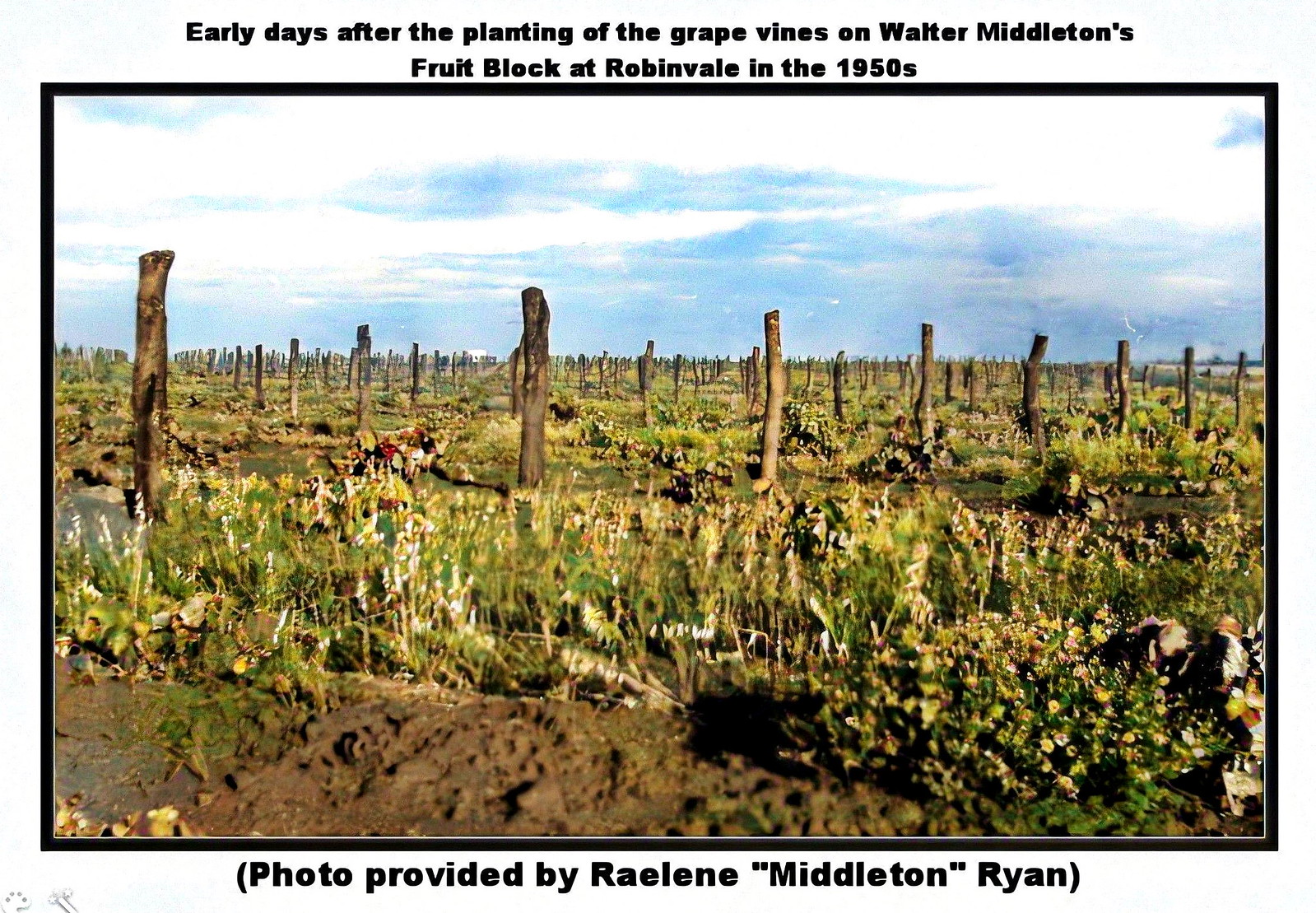This image features a historical photograph centered within a black border, documenting the early days after the planting of grapevines on Walter Middleton's fruit block at Robinvale in the 1950s. The photo, provided by Raylene Middleton Ryan, showcases a vast, muddy field lined with numerous wooden poles that stretch into the horizon. These poles were likely intended to support the grapevines as they grew. The land appears flat and barren in large patches but interspersed with some greenery, including grass and various plants, some of which have yellow and white flowers. The sky above is a clear blue with scattered clouds, adding contrast to the dry and rugged landscape below.